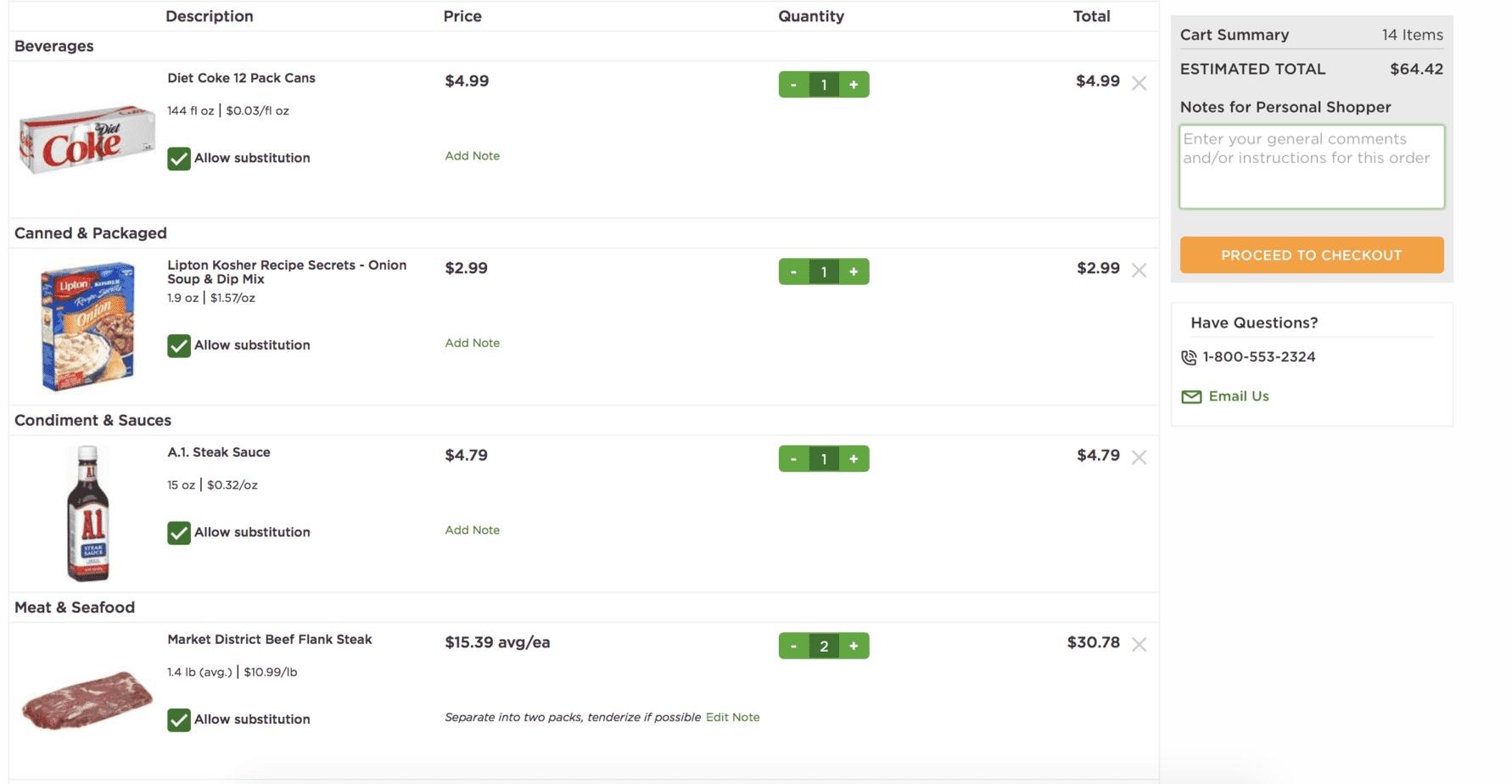The image captures a screenshot of a shopping cart summary from an online grocery website. The cart contains a variety of items:

1. **Beverages:**
   - **Diet Coke**: One 12-pack of cans priced at $4.99.

2. **Soups and Mixes:**
   - **Lipton Kosher Recipe Secrets Onion Soup Mix**: One package priced at $2.99.

3. **Condiments:**
   - **A1 Steak Sauce**: One bottle priced at $4.79.

4. **Meat and Seafood:**
   - **Market District Beef Flank Steak**: Two portions with a total cost of $30.78.

The cart summary indicates a total of 14 items, resulting in a subtotal of $64.42. At the bottom of the page, there is an orange "Proceed to Checkout" button with white text.